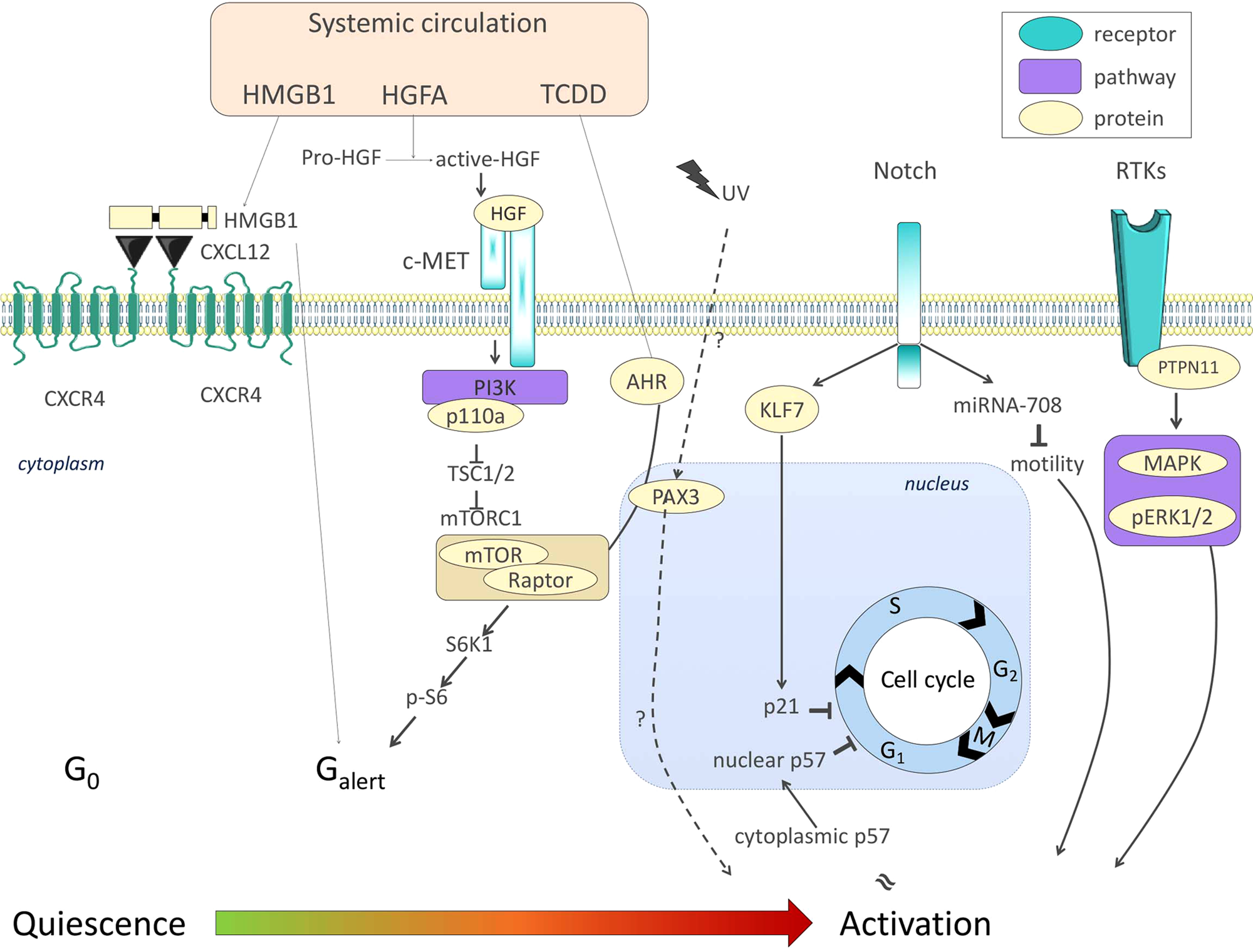The image is a scientific flowchart illustrating various cellular processes and their interactions. The chart features numerous graphics and text labels that identify different elements, starting from the left with terms like CXCR4, CXCR4, CXCL12, and HMGB1, followed by HGFA, and TCDD. A line descends to PRO-HGF, which then transitions rightward to ACTIVE-HGF. Below these terms, arrows lead to a circular label indicating HGF, and continuing with connections to elements labeled CMET, PI3K, P110A, TSC1-2, and MTORC1.

At the top left corner of the flowchart, a small beige box with black text denotes 'systemic circulation.' Throughout the diagram, various symbols represented in teal, purple, and yellow stand for receptors, pathways, and proteins respectively, as indicated by a legend in the upper right corner. The chart includes labels such as HMGB1, HGFA, and TCDD, which point to specific elements within the flowchart. Additionally, a prominent blue circle labeled with sections illustrates important details about the cell cycle.

Spanning the bottom of the image is a large arrow transitioning from green on the left, labeled 'quiescence,' to red on the right, labeled 'activation.' This gradient illustrates the progression from a dormant or resting phase to an active state within the cellular processes. The chart is set against a white background and presents a detailed, digitally created diagram that highlights the complexity of cell replication and growth, potentially relating to both human and animal cells. Blurred DNA or RNA sequences run across the top, further emphasizing the genetic context of the chart.